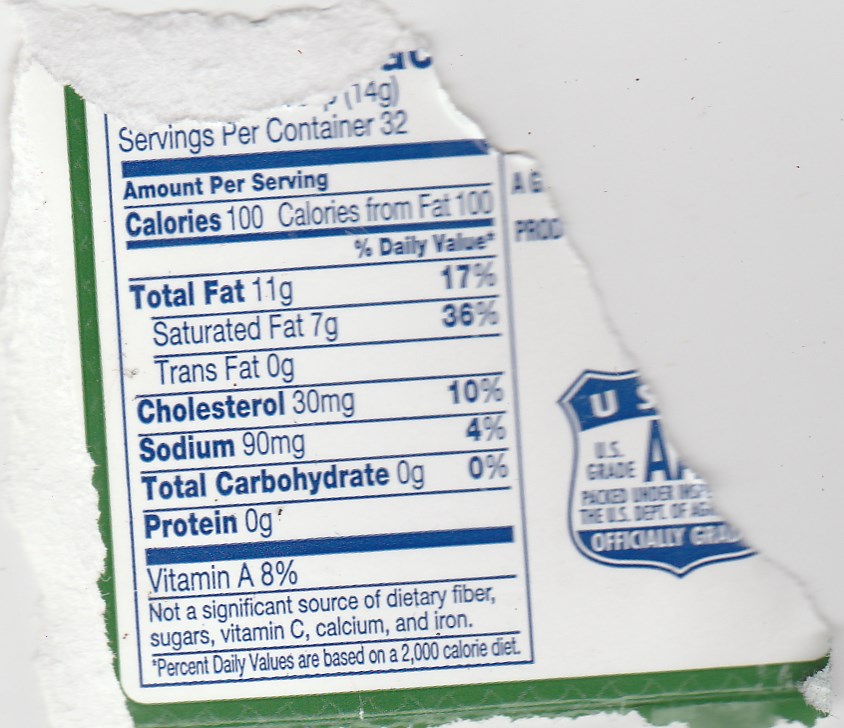The image depicts a close-up view of a torn piece of food packaging, specifically the nutrition label. The label, likely made of cardboard, is primarily white with a green border and features information printed in blue text. It lists essential nutritional details: servings per container are 32, with each serving amounting to 100 calories, all derived from fat. The total fat content is 11 grams (17% of the daily value), including 7 grams of saturated fat (36% of the daily value) and zero grams of trans fat. Additionally, the cholesterol content is 30 milligrams (10% of the daily value), sodium is 90 milligrams (4% of the daily value), and both total carbohydrates and proteins are absent. The label notes 8% Vitamin A, with an indication that it is not a significant source of dietary fiber, sugars, Vitamin C, calcium, or iron. A partially visible seal mentions "USDA officially graded," further adding to the authenticity and regulatory compliance of the packaging.